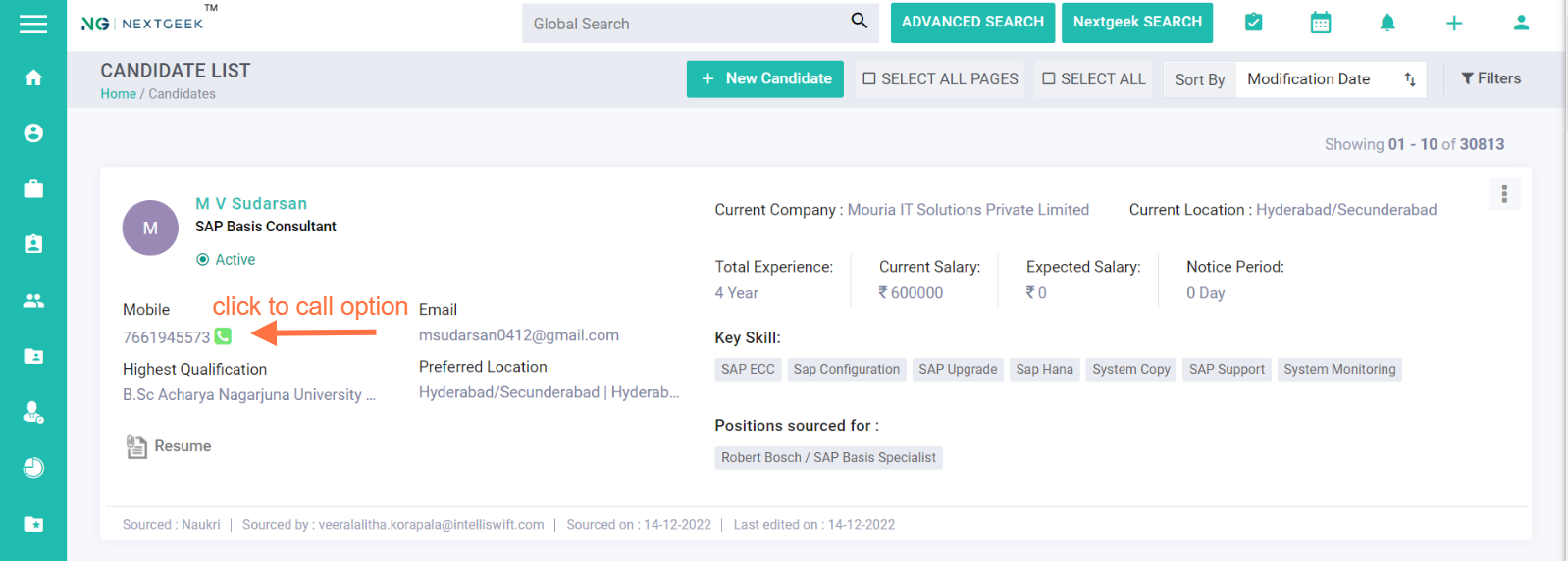This image is a screenshot from the website "NextGeek." In the upper left-hand corner, the "NextGeek" logo is displayed with the "NG" symbol to its left. A vertical menu runs along the entire left side of the screen. To the right of the NextGeek logo, there's an expansive gap, followed by a global search bar. Adjacent to the global search bar is a green "Advanced Search" button. Next to this is a "NextGeek Search" button. Moving further right, there are five icons.

On the next row down, the text "Candidate List" appears on the left, indicating that the user is on the "Candidates" page of the website, navigated from the home page. To the right, within the same line, is an "Add New Candidate" button featuring a white "New Candidate" label and a plus sign for adding new candidates.